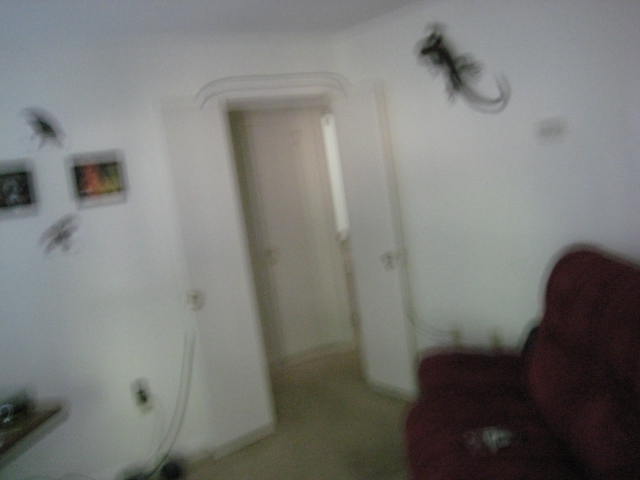In this slightly blurry photograph of what seems to be the interior of a house or apartment, we observe white walls and a red or burgundy couch positioned in the lower right-hand corner. Hanging on the walls are a couple of square pieces, likely serving as wall art. The most intriguing aspect of the photo is the outline of a lizard on the right wall, accompanied by the outlines of additional creatures on the left wall. The outlines appear to be decorative rather than real, adding an element of curiosity to the otherwise ordinary indoor setting.